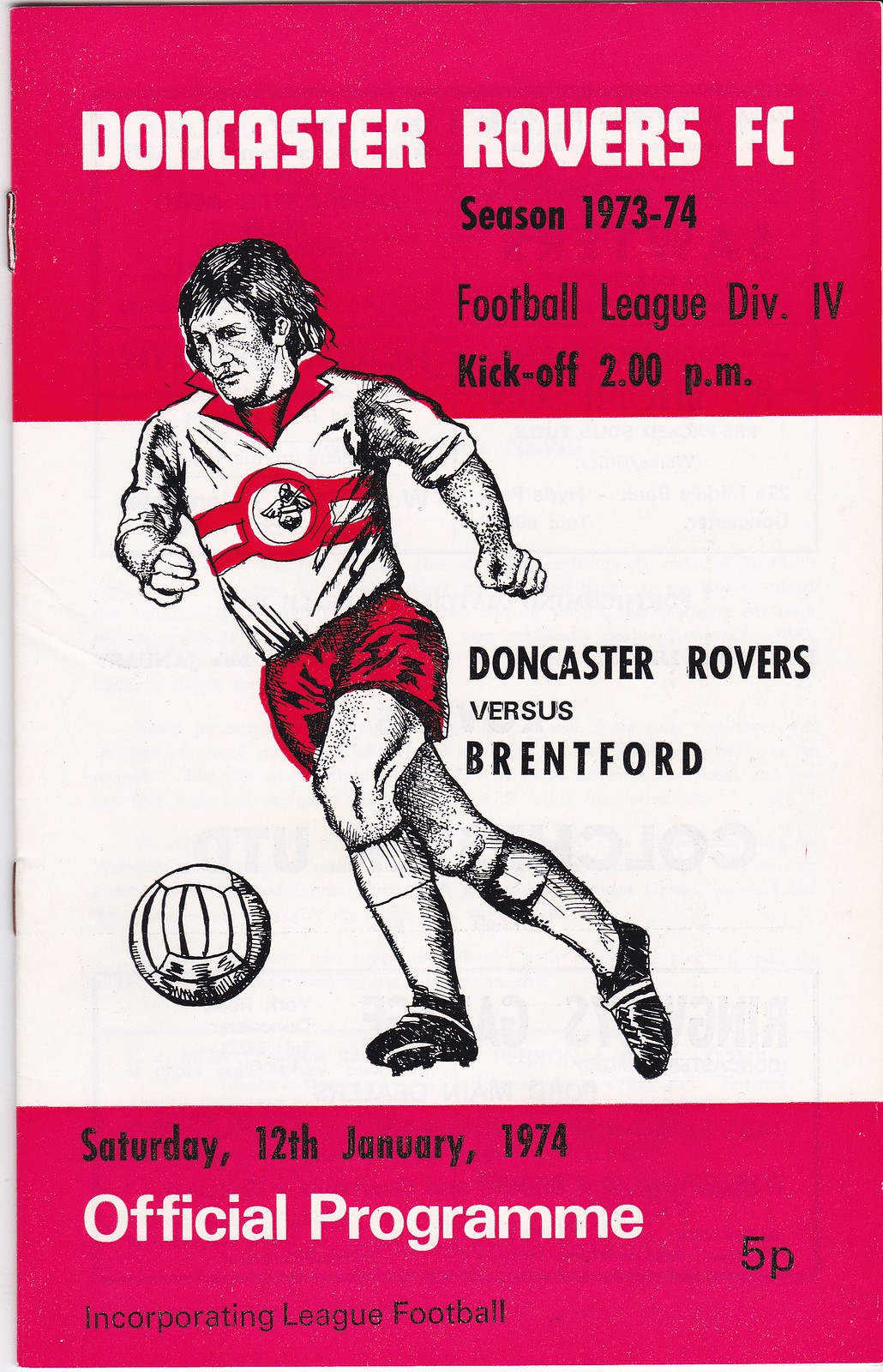This is a vintage soccer program cover for the Doncaster Rovers FC 1973-74 season, specifically for their Football League Division IV fixture against Brentford. The background features a red-white-red color scheme from top to bottom. Central to the design is an artist’s depiction of a player in motion, dressed in the Doncaster Rovers’ white and red kit, with red shorts, mid-stride as he prepares to kick an all-white ball. The player's detailed shaggy hair adds to the dynamic feel of the illustration. Above the player, white lettering reads: "Doncaster Rovers FC." Directly below, it states: "Season 1973-74, Football League Division IV, Kickoff 2pm." To the right of the player, it announces: "Doncaster Rovers vs. Brentford." At the bottom, within the red section, it details: "Saturday, 12th January 1974, Official Program Incorporating League Football," and the price, "5p." Two visible staples secure the edge of the booklet, completing the classic look of this nostalgic sports memorabilia.